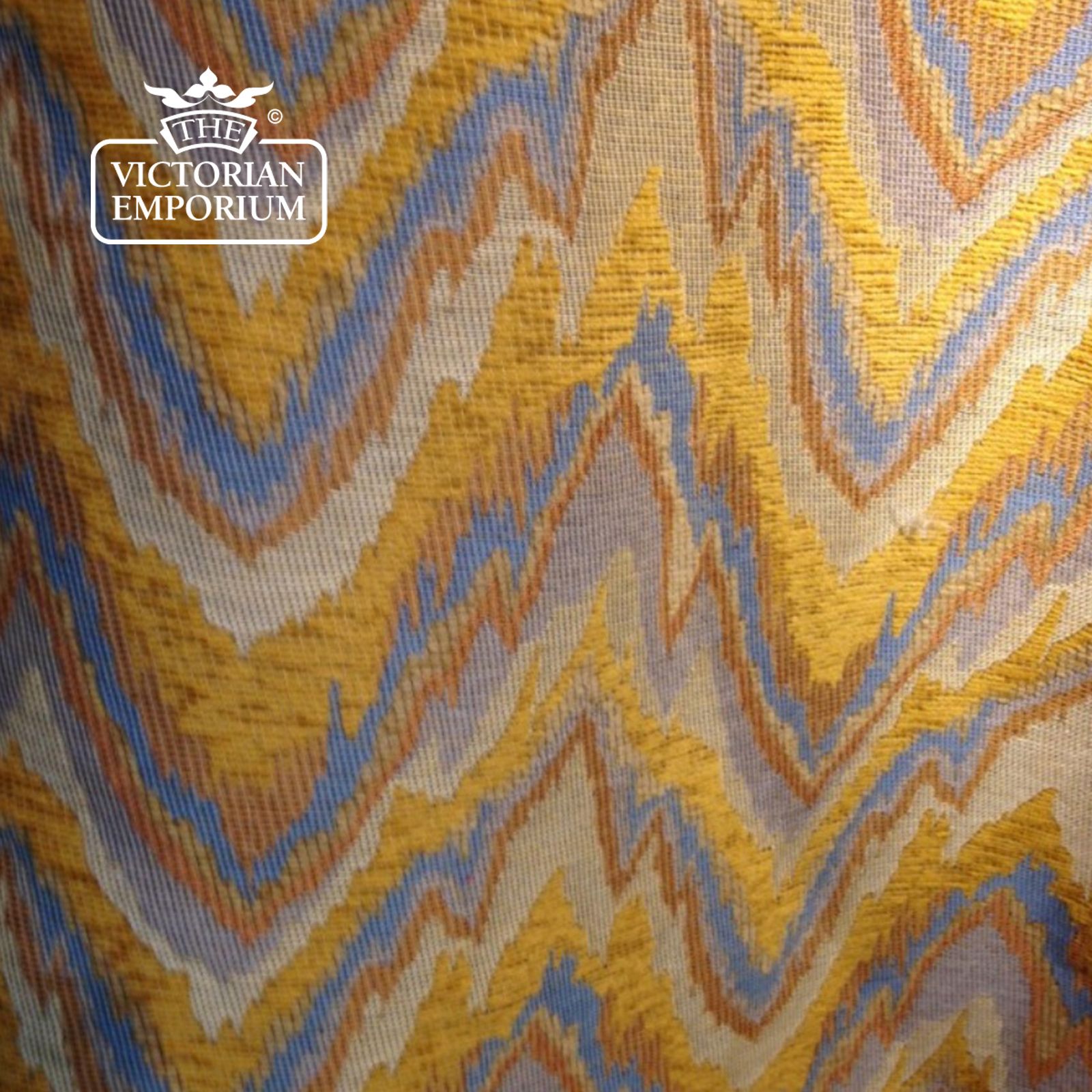The image displays a detailed close-up of what appears to be a textile, possibly a woven tapestry or a fabric throw. The textile features a repeating pattern of wavy, mountain-like craggy shapes in vibrant colors including off-white, orange, blue, yellow, and gray. The gold sections of the pattern are notably thick and raised, adding a textured dimension to the material.

In the upper left corner, there is a bold overlay or watermark displaying a white rectangular logo with curved corners. Inside the rectangle, the text reads "Victorian Emporium" in white letters. Above this text is a small banner with the word "The" and a three-leafed shape with leaves extending to the left and right. There is also a "C" enclosed within a circle. The overall image is brightly lit with clear visibility of the intricate details and vibrant hues of the fabric.